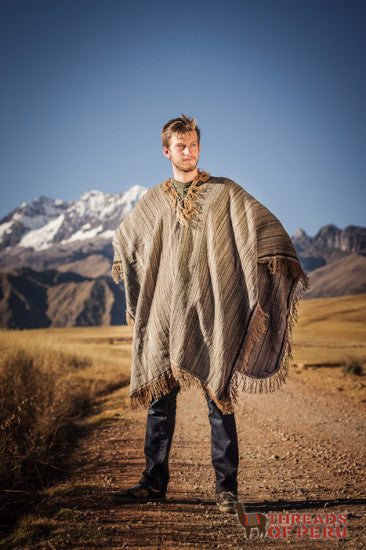In this vertical rectangular image, a young man stands in a mountainous area, framed against a backdrop of towering peaks and a strikingly blue sky. His light, slightly tousled hair and modest beard around his chin give him a distinctive look. He is wearing jeans and boots, complemented by a draped brown poncho with fringe, similar to a blanket with a hole cut out for his head. The ground beneath him is bare, brown dirt. In the background, snow-capped gray peaks rise sharply, suggesting a dramatic drop-off behind him. The sky above transitions from a darker blue at the top to a lighter shade closer to the horizon. To the bottom right of the image, there is an artwork of a brown llama with the words "Threads of Peru" written in red next to it, adding a cultural element to the scene. The man gazes off to the right, his attire and stance reflecting a fusion of ruggedness and traditional style.